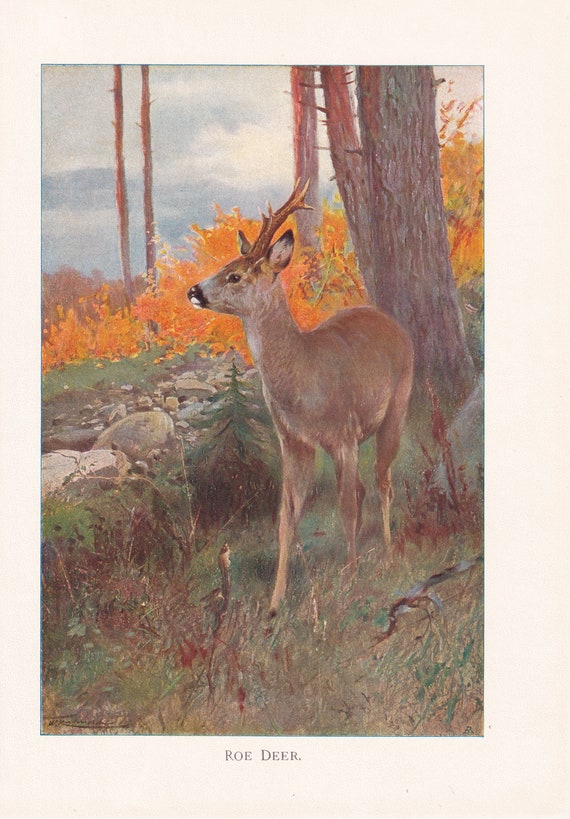The painting captures a majestic Roe Deer buck standing alone in the tranquil scenery of a forested hillside. The forest is vibrant with bright yellow and orange shrubbery, narrow saplings, and a prominent large tree behind the deer. The setting evokes a sense of wilderness with various natural elements like green underbrush, low-growing pine trees, scattered branches on the forest floor, and a smattering of rocks. The buck, a six-point deer with three points on each antler, is depicted in a slightly sideways stance, showcasing only the left side of its face. Its horns are tall and branch elegantly, while the deer's brown fur and black nose contrast beautifully against the bright and earthy colors surrounding it. In the background, a mountainous landscape disappears into a cloudy, gray-blue sky. There is a soft pink border framing the image, adding a gentle touch to the natural setting. Additionally, a bird is subtly present in the picture, enhancing the overall vibrancy of the outdoor scene. At the bottom of the artwork, the title "Roe Deer" is inscribed, emphasizing the subject of this serene and detailed depiction of nature.